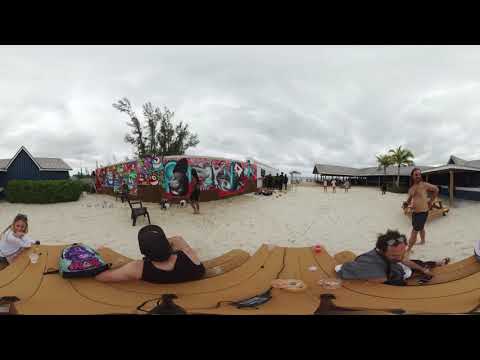This panoramic beach photograph features a dynamic yet serene scene under a very cloudy, gray sky, hinting at impending rain. The central focus is on a pair of brown, semi-circled benches on the sand. Seated back-to-back on the benches are two people: a man with sunglasses on his forehead and a woman in a white long-sleeved shirt. Next to them sits another woman in a black bathing suit with a bag resting on her elbow. A lone, empty seat sits in front of this woman, accentuating the openness of the surroundings. 

In the backdrop, a vivid red fence adorned with numerous murals stretches across the left side of the picture, giving the appearance of vibrant yet controlled graffiti. To the right side of the image stands a blue building, possibly a restroom, bordered by a green hedge and partially obscured by a palm tree. Further right, a covered area, likely a restaurant with tables, houses more people. A man in a bathing suit strolls on the sandy beach toward the center of the photo, adding life and movement to the tranquil setting. 

Additionally, the photo is framed by black borders at the top and bottom, with the clouds just below the upper border, enhancing the rectangular composition and emphasizing the overcast ambiance of the scene. The setting, while serene, evokes a sense of community and activity, with people milling about and engaging in their beachside routines.